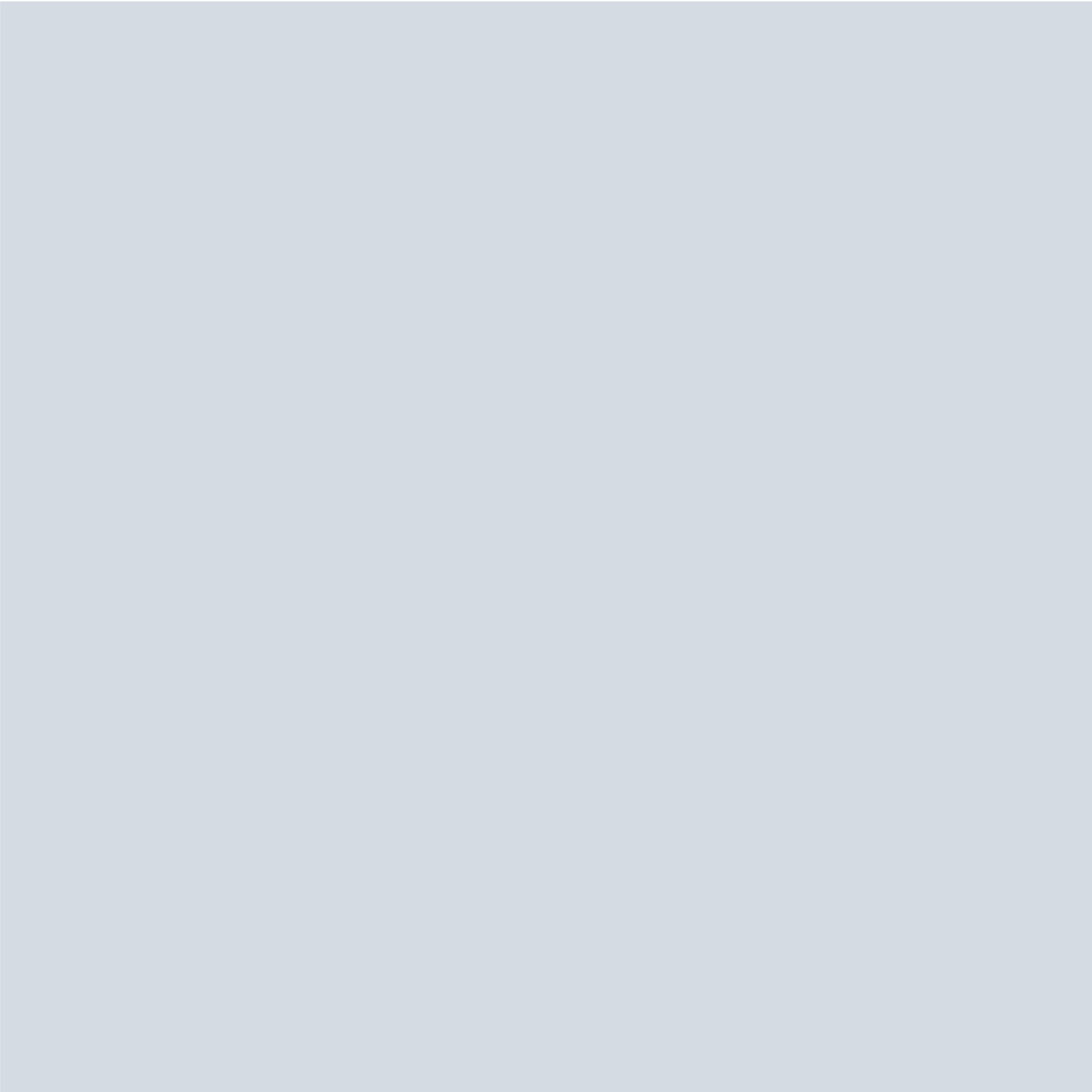A minimalist square image with a perfectly solid color fills the frame. The hue is a light gray with a subtle blue tint, creating a very pale, bluish-gray or grayish-blue color, depending on your perspective. The image has no other details, patterns, or textures—just an uninterrupted expanse of this soft, monochrome shade. The dimensions are perfectly symmetrical, balancing height, width, and length into a harmonious square. No hidden elements, secret messages, or any form of variation exist within this simple, uniform composition. The image stands as an exercise in minimalism and color perception, challenging the viewer to find depth and interest in its stark simplicity.